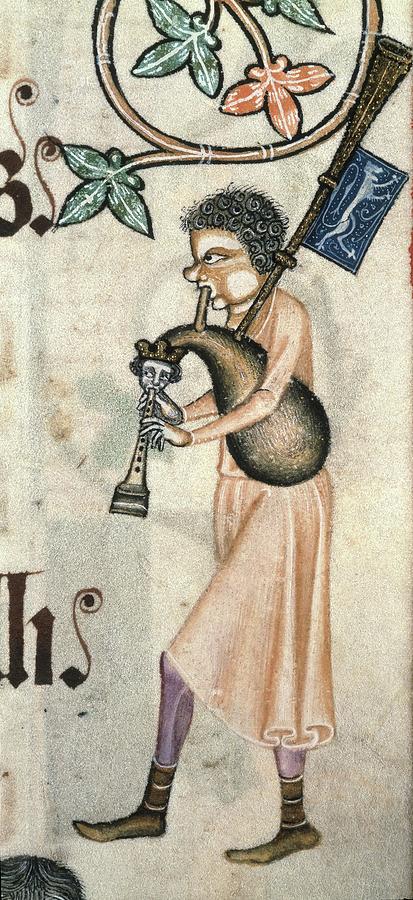The image is of a detailed medieval-style tapestry or rug featuring a person playing a bagpipe-like instrument. The person, with exaggerated features and short curly hair, is depicted in a light, almost dull pink gown, along with purple leggings or legs and brown high-top, slipper-like shoes. The bagpipes include a notable clarinet portion that has a small man's head seemingly playing it. A blue banner featuring a stylized lion or large feline, reminiscent of ancient rock drawings, is attached to the elevated pipe of the bagpipes. Above the person's head is a floral vine design with green and red leaves formed into a circle. The scene is set against a cream-colored background, and there are partially visible, unreadable letters to the left.